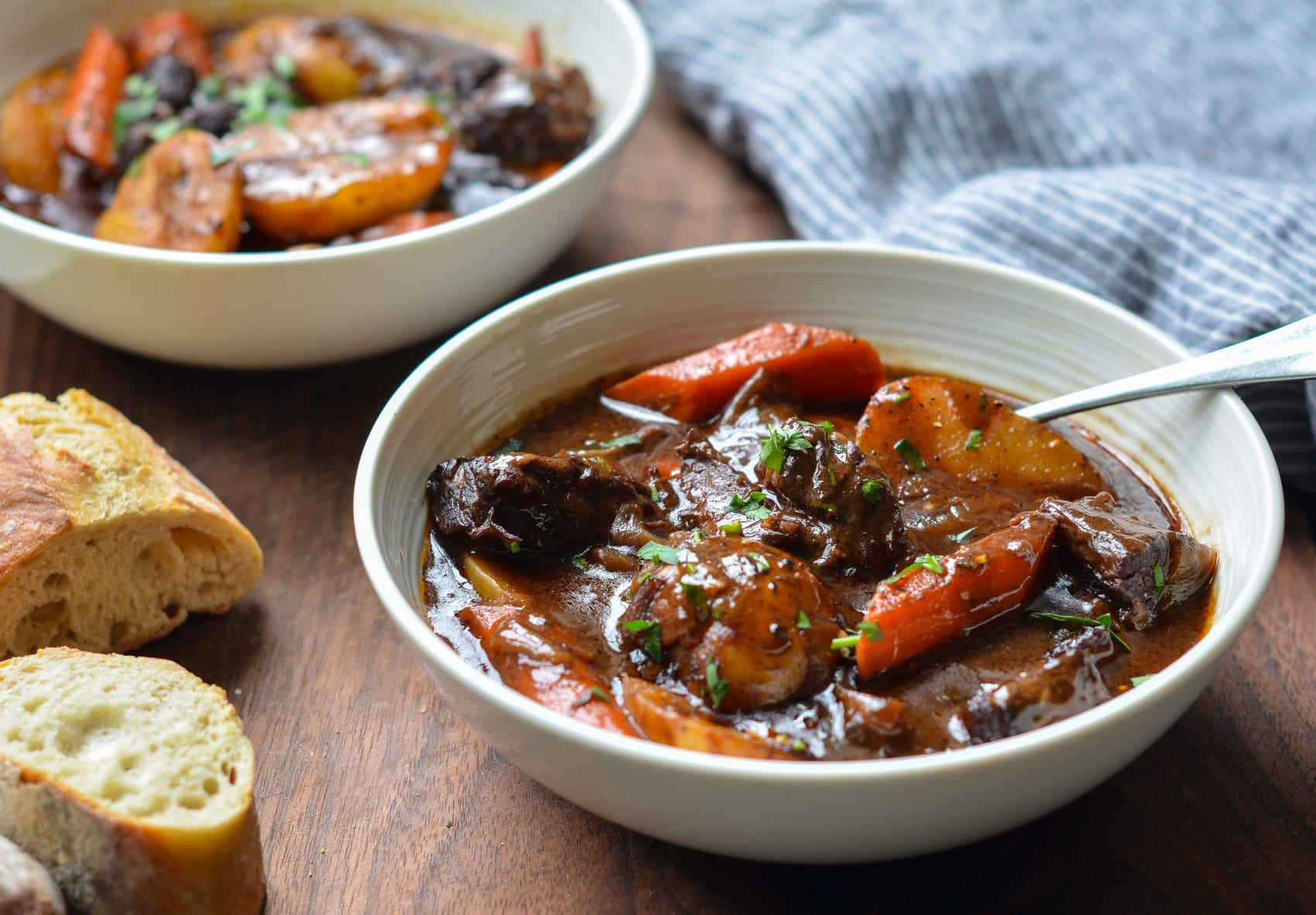This detailed photograph captures two white bowls, each filled halfway with a hearty beef stew, set upon a wooden table. The stew features large chunks of beef, potatoes, and carrots, with a sprinkle of green herbs—possibly cilantro or parsley—adding a touch of color on top. The stew itself has a rich, brownish-red hue, complemented by occasional hints of tomatoes. One bowl includes a spoon partially obscured by the contents, while the other bowl lacks any utensils. In the lower left-hand corner of the image, two pieces of French baguette, about two inches each, lay cut-side up, potentially buttered. A neatly folded blue and white striped cloth napkin adorns the upper right quadrant of the scene, enhancing the rustic and inviting atmosphere.